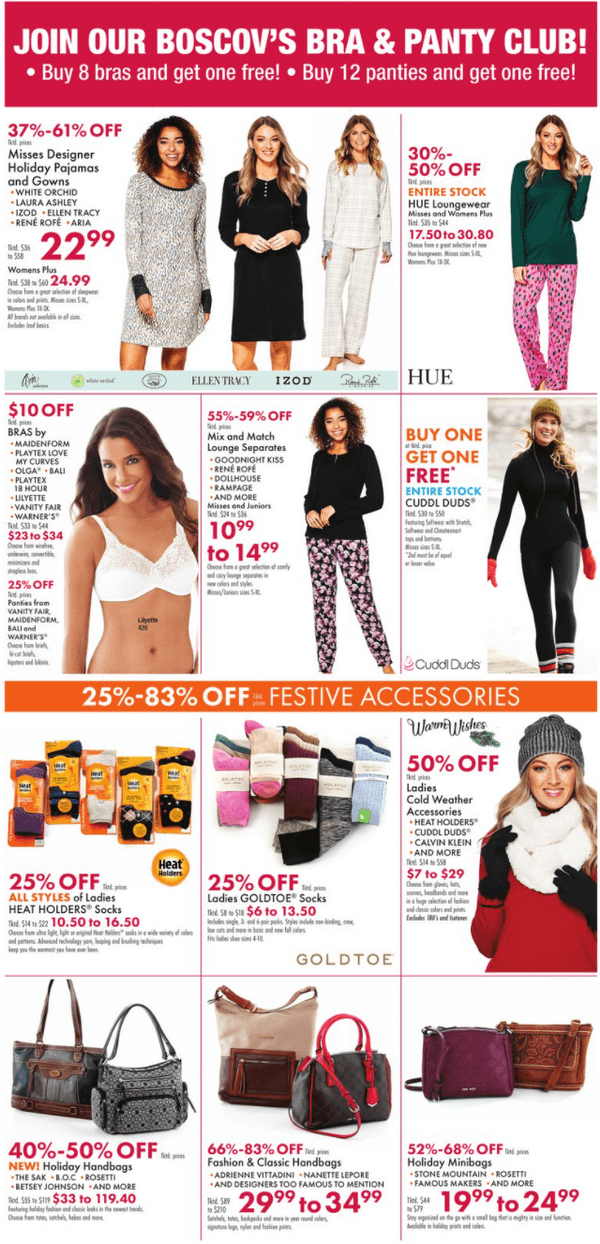**Detailed Caption:**

The image is from an online page promoting Boscoff's clothing and accessories. A vibrant red banner spans the top, inviting customers to join Boscoff's Bra and Panty Club with an enticing offer: "Buy eight bras and get one free. Buy 12 panties and get one free."

Directly beneath the banner is a photograph of three women clad in cozy pajamas, accompanied by text that reads: "Mrs. Designer Holiday Pajamas and Gowns" priced at $22.99. Adjacent to this, on the right, another woman showcases stylish loungewear with detailed information about the product, including its sale and pricing.

Moving below, on the left, a woman is seen wearing a white bra. Next to her is detailed information concerning the available bras along with their pricing. To the right of this image sits another photo of a woman in different loungewear. Accompanying this, text provides specifics about the ongoing sale, prices, and product details.

On the far right, a woman is depicted outdoors in winter attire with a promotional message: "Buy one, get one free." Below these images are additional photos targeting winter essentials. The first depicts winter socks, marked with "25% off" below it. Adjacent is a collection of women's socks in various colors.

Further to the right, a woman is featured wearing a winter hat, scarf, and gloves. Below this, a series of pictures display handbags: two purses on the left, three in the center, and two smaller purses on the far right.